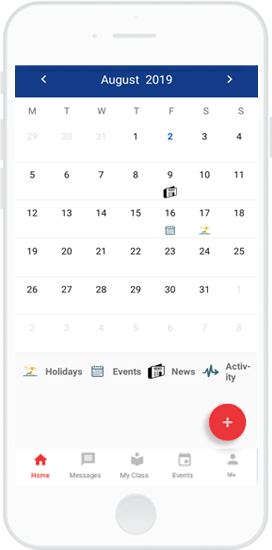The image is a detailed screenshot of a phone calendar for August 2019, featuring a clean white background. At the very top center of the screen, a thin gray line spans horizontally. Directly below this line, a cobalt blue rectangle stretches from left to right, containing white text and directional arrows. The arrow on the left points leftward, the arrow on the right points rightward, and the text in the center reads "August 2019."

Just below this blue bar, a row displays the days of the week, starting with Monday and ending with Sunday. The calendar days begin on a Tuesday (the 1st of August) and conclude on a Saturday (the 31st). Noteworthy dates include the 9th, 16th, and 17th, each marked with unique icons that likely indicate events, holidays, or news.

Further down, there is a legend explaining the icons: holidays are represented first, followed by a small calendar for events, a partial newspaper for news, and an up-and-down graph for activity.

Towards the bottom right of the screen, a red circle with a white plus sign at its center invites the user to add new entries. Finally, an icon bar spans from left to right at the bottom of the screen, featuring options labeled as Home, Messages, My Class, Events, and Me.